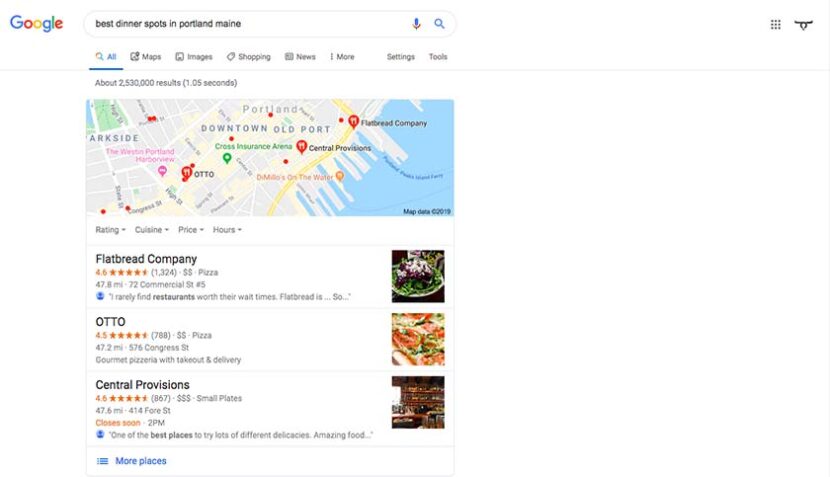The image shows Google search results for "Best dinner spots in Portland, Maine" entered into the search bar. The search is set to "All" and "Open now." At the top, there's a map with three locations marked. Below the map, the following restaurants are listed with detailed information:

1. **Flatbread Company** – Rated 4.6 stars from 1,324 reviews, this restaurant is categorized with two dollar signs ($$). It specializes in pizza and is located at 72 Commercial Street. Notable comment: "I rarely find restaurants worth their wait times. Flatbread is so..."

2. **Otto** – With a rating of 4.5 stars from 788 reviews, Otto also falls under the two dollar signs category ($$). This pizza place offers gourmet pizza with takeout and delivery options. It is situated at 576 Congress Street.

3. **Central Provisions** – This establishment boasts a rating of 4.6 stars from 867 reviews and is marked with three dollar signs ($$$). Known for its small plates, it is located at 4144 Street and closes soon at 2 p.m. Highlighted review: "One of the best places to try lots of different delicacies, amazing food."

Each listing features a thumbnail image on the right, displaying vibrant colors including red, blue, white, yellow, black, orange, pink, and brown.